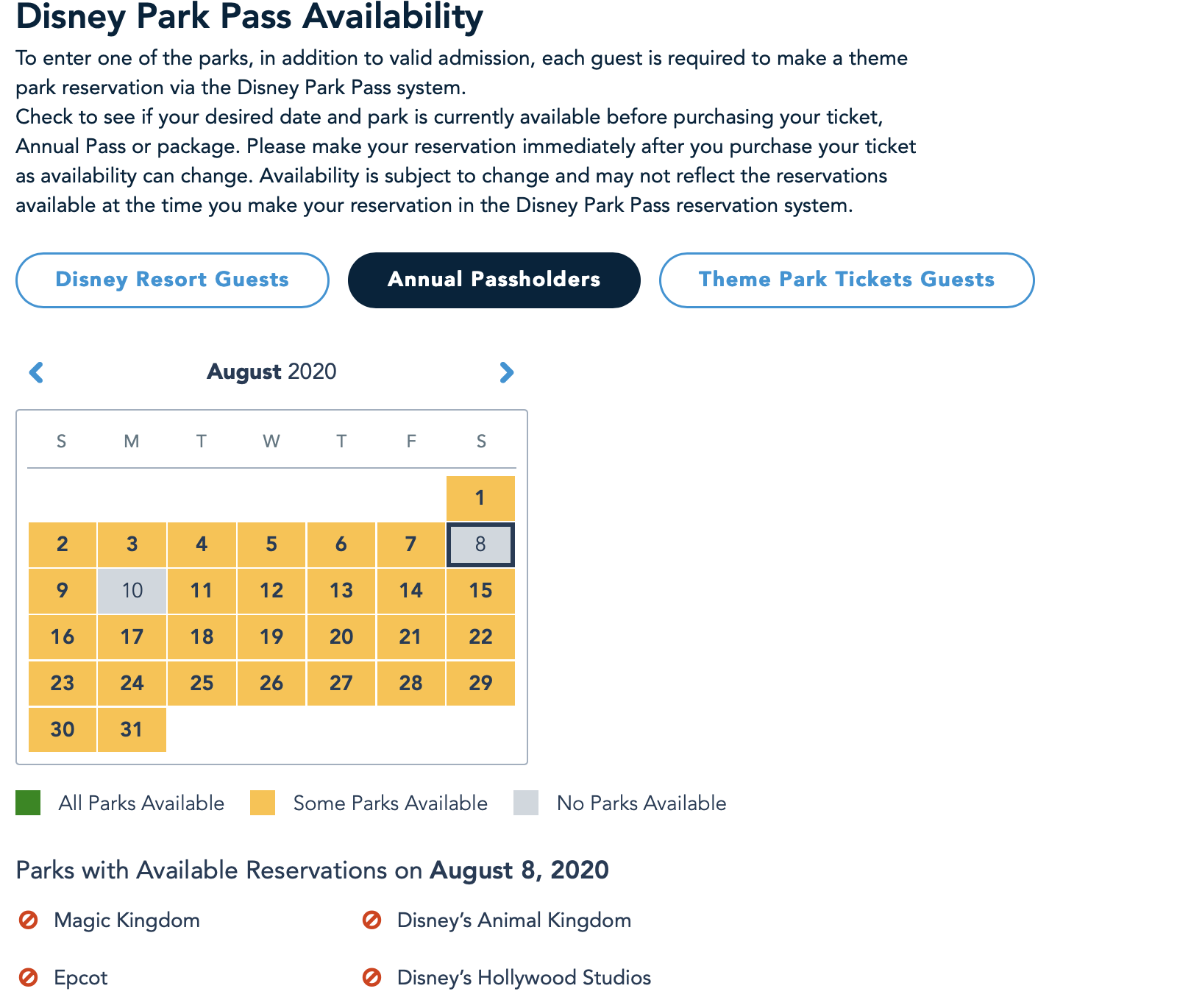### Detailed Caption:

The image is a detailed screenshot of the "Disney Park Pass Availability" screen, prominently displayed in bold black letters at the top. Below this headline, a notice explains the requirement for theme park reservations: "To enter one of the parks, in addition to valid admission, each guest is required to make a theme park reservation via the Disney Park Pass system. Check to see if your desired date and park are currently available before purchasing your ticket. For Annual Pass or Package holders, please make your reservation immediately after purchasing your ticket as availability can change." It also notes that "Availability is subject to change and may not reflect the reservations available at the time you make your reservation in the Disney Park Pass reservation system."

The notice caters to three categories of visitors: "Disney Resort Guests," "Annual Pass Holders," and "Theme Park Ticket Guests." The "Annual Pass Holders" category is highlighted in black, while the other two categories are highlighted with white text on a blue background.

A calendar interface for August 2020 is displayed, allowing users to adjust dates and times. Notably, August 8th and August 10th are marked in gray, with the 8th having a distinct black trim around its box, indicating it is the selected or hovered date. Other dates are marked in gold.

At the bottom of the screen, a color code explains park availability: "all parks available" in green, "some parks available" in gold, and "no parks available" in gray. According to the calendar, for August 8th, 2020, all four Disney parks—Magic Kingdom, Epcot, Disney's Animal Kingdom, and Disney's Hollywood Studios—have available reservations.